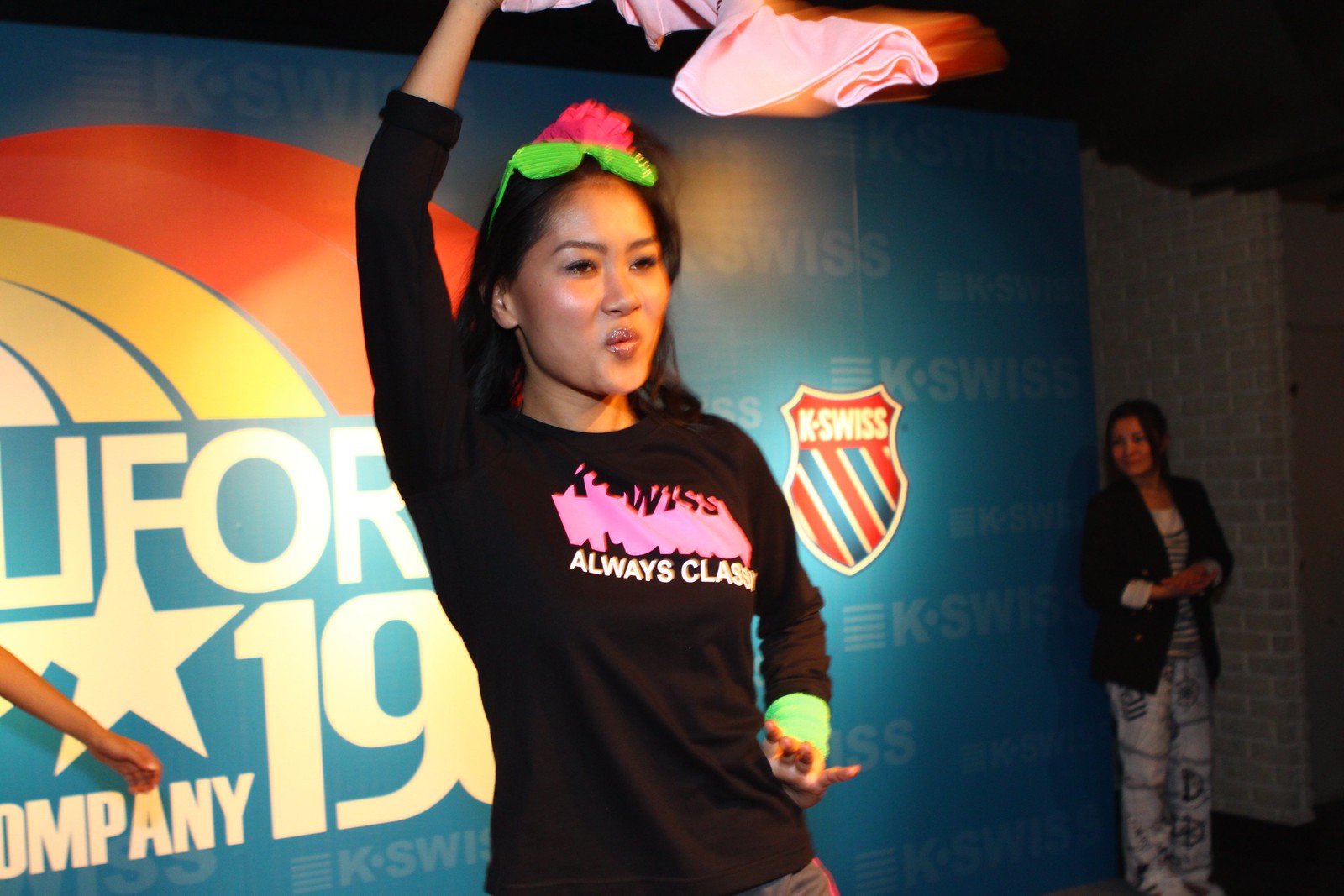The photograph captures a dynamic scene with a woman at its center, seemingly dancing. She is waving a pink piece of cloth with her right hand, while her left hand rests on her hip. The woman is sporting a long-sleeved black t-shirt emblazoned with the words "ALWAYS CLASSY" in white text. Her head is adorned with green shutter shades, reminiscent of the "Kanye West" style, and a red flower. Her black hair cascades down to her shoulders. 

She stands in front of a solid blue board, partially obscured by her figure, with legible letters that spell out "F-O-R," followed by a star, "1-9," and "M-P-A-N-Y." To the right side of this board is a prominent SHIELD logo featuring blue, white, and red lines, topped with the text "K-Swiss" in white. 

The background also hints at additional elements such as a gray brick wall on the far right and a black top section, adding layers to the image. Additionally, another woman can be seen looking on; she is dressed in a black blazer over a white blouse paired with blue jeans. Combining these details, the image vividly portrays a lively and colorful moment frozen in time, with the dancing woman as the captivating focal point.